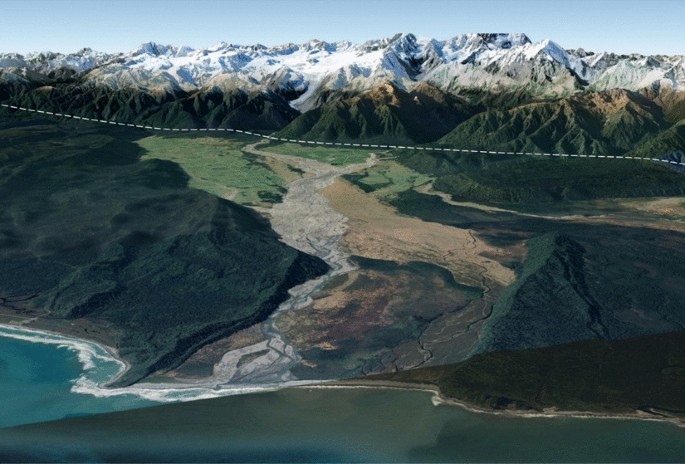The image captures an expansive natural landscape, starting from a serene shoreline at the bottom where white surf meets the beach. Above the shore lies a body of water, transitioning into a hilly area adorned with various shades of green vegetation. Central to the landscape is a creek meandering through the hills, flanked by patches of reddish-brown and light brown terrain, indicating areas with scarce vegetation. On the left, a large swath of olive green contrasts sharply with the other greens. A distinct white dashed line runs horizontally at the base of a range of green hills, which gives way to higher, snow-capped mountains in the distance. Crowning the scene is a narrow strip of clear blue sky, completing this tranquil and picturesque outdoor view.